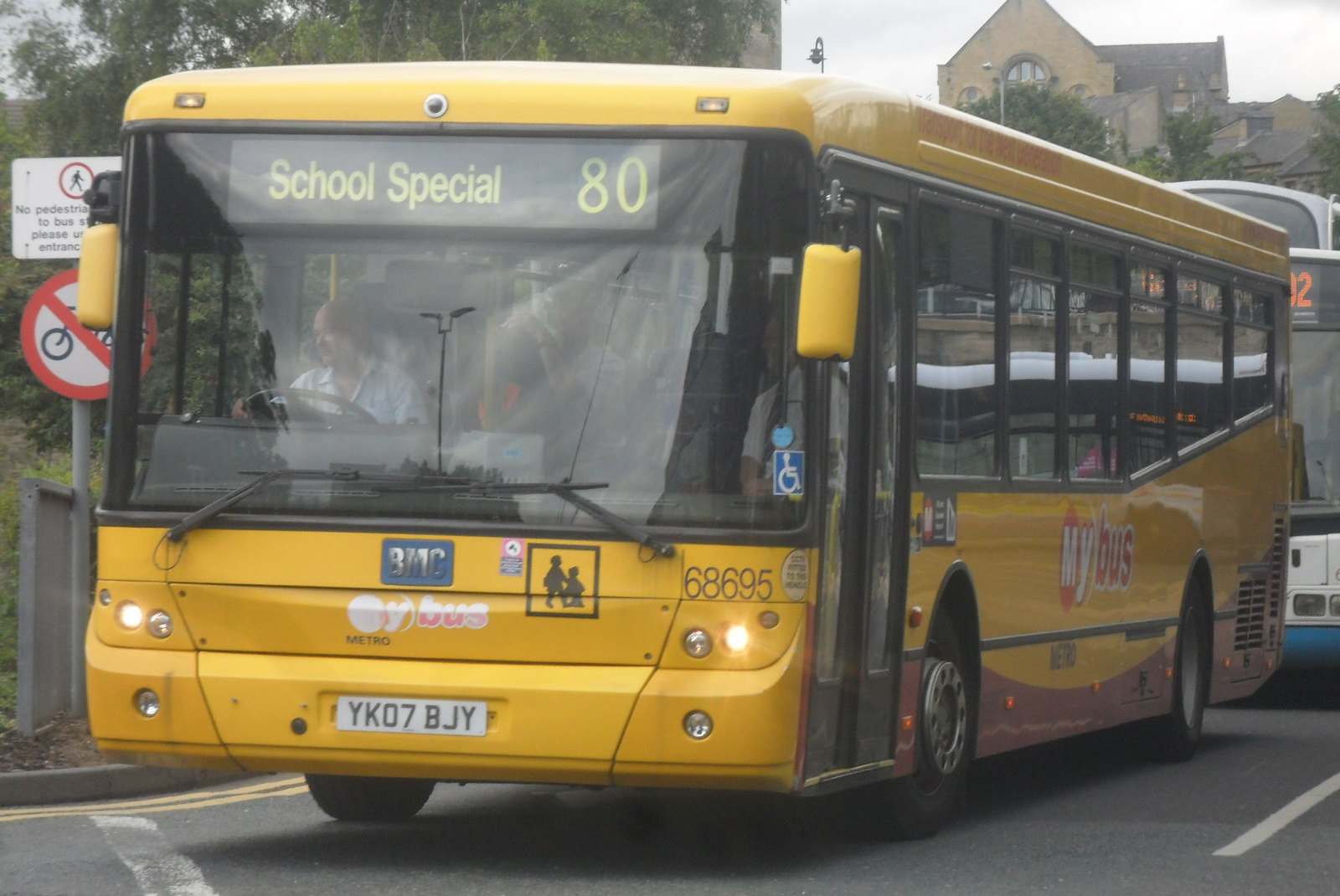In this photograph, a yellow school bus labeled "School Special 80" is prominently displayed as it makes a right-hand turn on an asphalt road. The bus, manufactured by BMC, features "my bus" on its sides, with "my" in white letters and "bus" in red. The license plate reads YK07 BJY. A person is visible near the entryway, waiting to disembark. Behind the yellow bus, there is a blue, white, and black public transit bus with a partially visible digital banner. Road markings and a "No Bicycles" sign with a red slash are visible on the right side of the road. The background features a couple of trees, buildings on the upper right, and a cloudy sky. The scene appears to be set in a city during the daytime, likely captured from the perspective of another vehicle on the road.